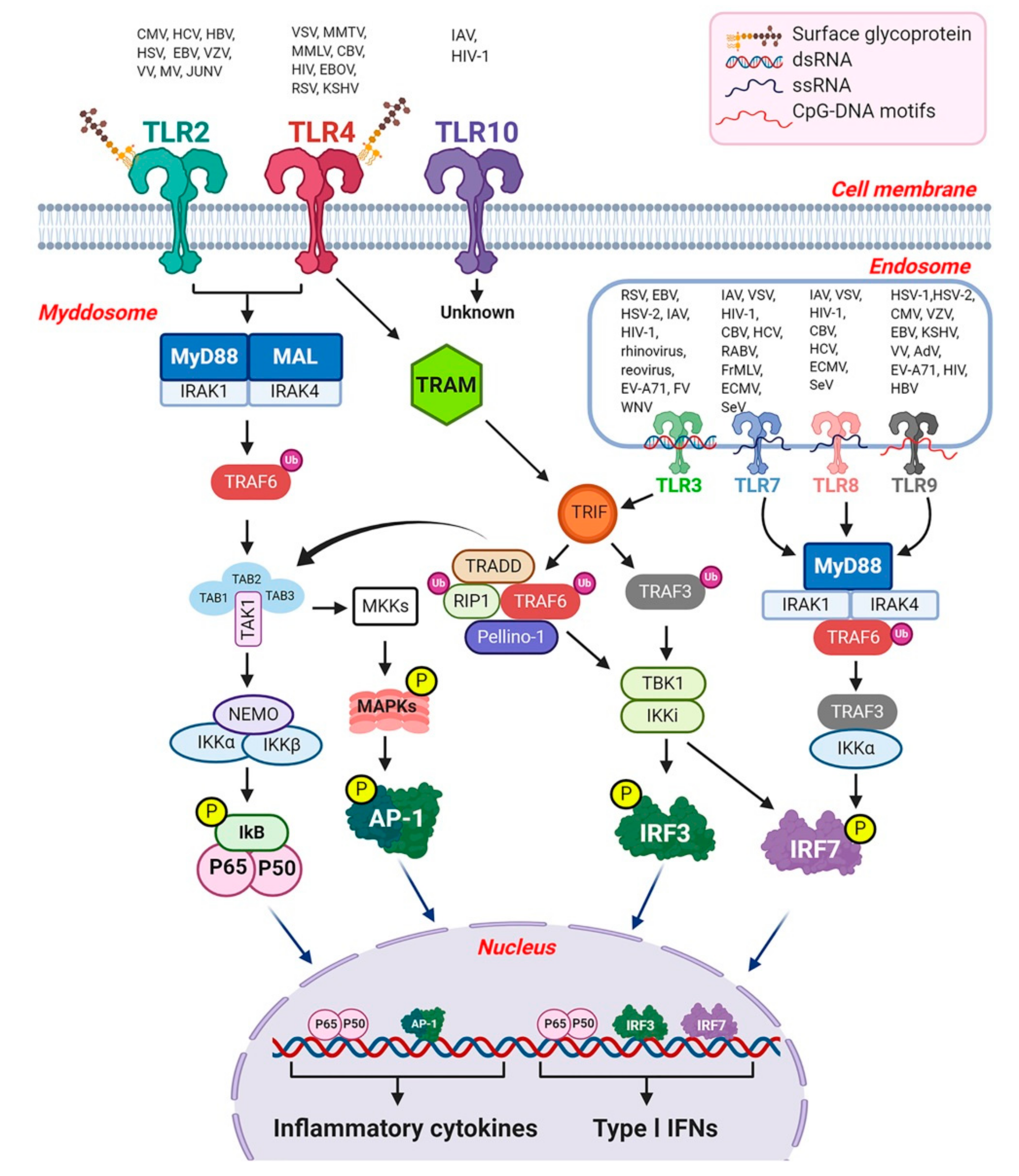The image presents a detailed and multicolored medical flowchart, illustrating the complex signaling pathways of Toll-Like Receptors (TLR), particularly focusing on the proteins activated once a ligand binds to a TLR receptor. The chart appears highly technical with various icons and symbols, highlighting components such as cell surface glycoproteins, DSRNA, SSRNA, and CPG-DNA motifs. Progressing from top to bottom, the chart maps out the signaling cascade starting from the cell membrane through intermediates like TLR2, TLR4, TLR10, and various endosomal pathways, including TRAF6, TAC1, NEMO, TRAM, TRIF, leading to inflammatory cytokines within the nucleus. Black arrows guide the flow between multicolored tabs labeled with different combinations of letters and numbers (e.g., Type 1 IFNS). The left side delineates an almost family tree-like structure of these interactions, emphasizing the intricate nature of intracellular communication and protein phosphorylation events within cellular immune responses.